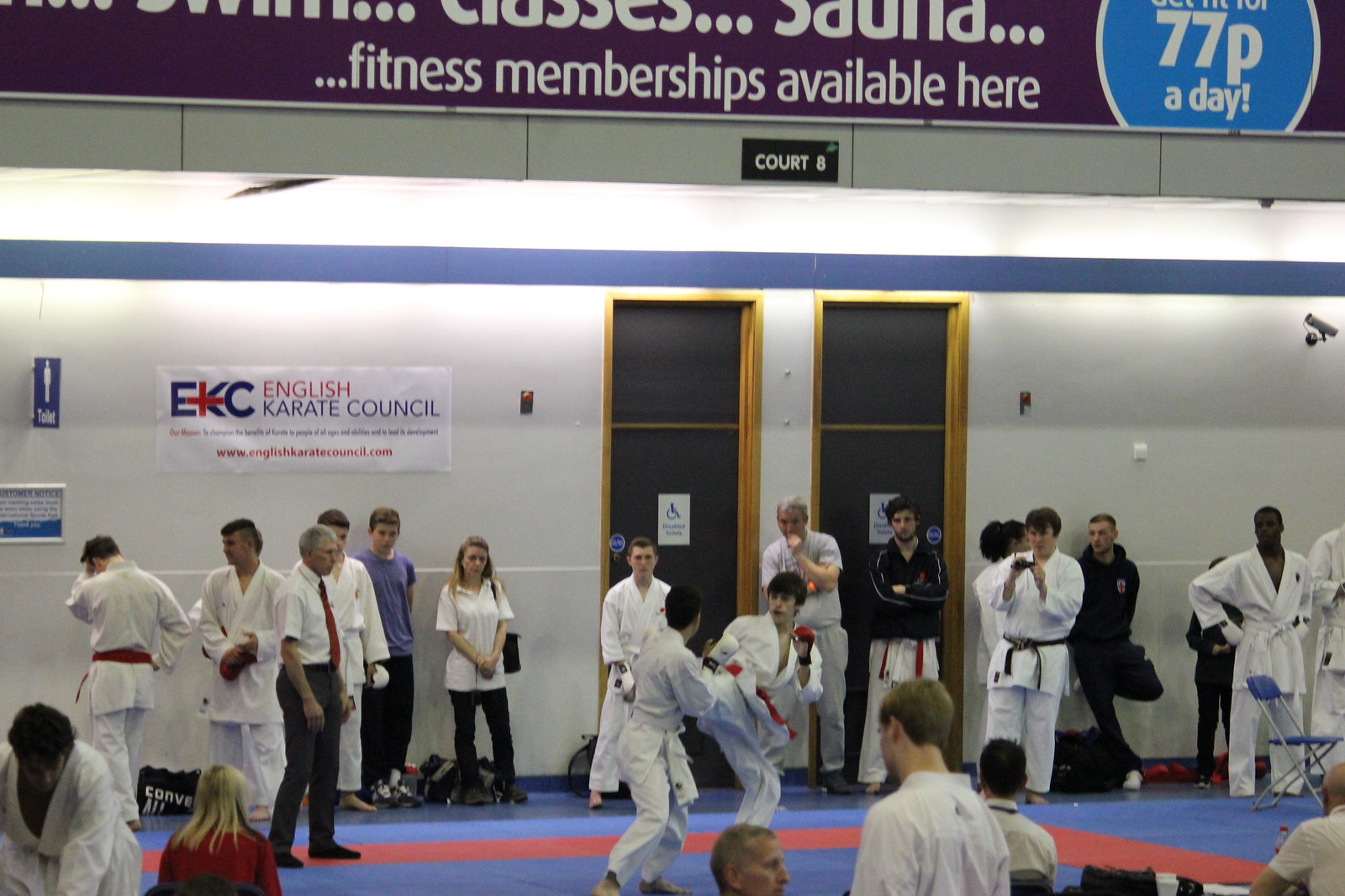This photograph captures a lively scene inside a karate dojo or studio with high ceilings and white walls adorned with a promotional banner and a poster from the English Karate Council. The floor features a bright blue mat with a red border, designating the sparring area where two older boys are actively engaged in combat, with one executing a kick towards his opponent. Surrounding the sparring area, numerous participants clad in traditional white karate gis with belts of various colors—red, black, and white—stand alongside coaches and spectators dressed in everyday clothing. The audience members, interspersed around the room, keenly observe the matches, contributing to the dynamic atmosphere of the tournament or class in session.